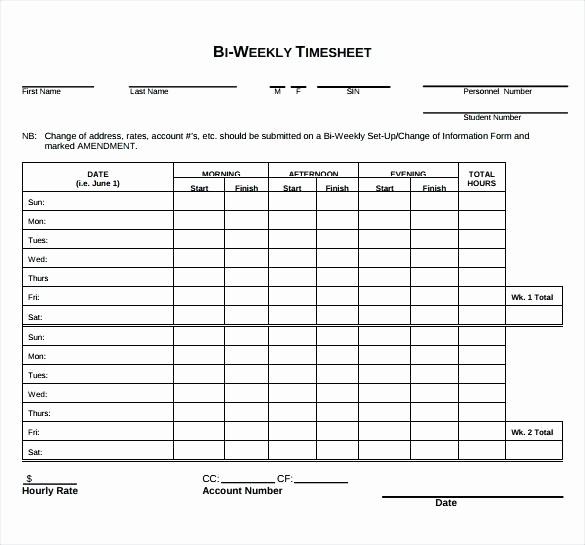The image is a detailed black-and-white scanned photocopy of a bi-weekly timesheet. The headline "Bi-Weekly Timesheet" is prominently displayed at the top. Below it, there are several fields for personal information, including lines to fill out the first name, last name, social security number (labeled as SIN), personnel number, and student number. There is also a field for indicating gender (M or F) and a note regarding change of address, rates, account numbers, and amendments, which should be submitted on a separate biweekly form.

The timesheet is divided into two sections, each representing a week. Each day of the week, from Sunday to Saturday, is listed with corresponding columns for the date, morning, afternoon, evening, start and finish times, and total hours worked. At the bottom of each week's section, there are rows to record the weekly totals. The form mentions using fields to record hourly rates and includes instructional text, such as "NB" for noting important changes.

The overall design of the timesheet is highly structured and organized, with all elements correctly aligned and centered. Fonts used include a prominent copperplate Gothic for headings and Helvetica for the remaining text, emphasizing a traditional office document style meant for employees to fill out their work hours systematically.